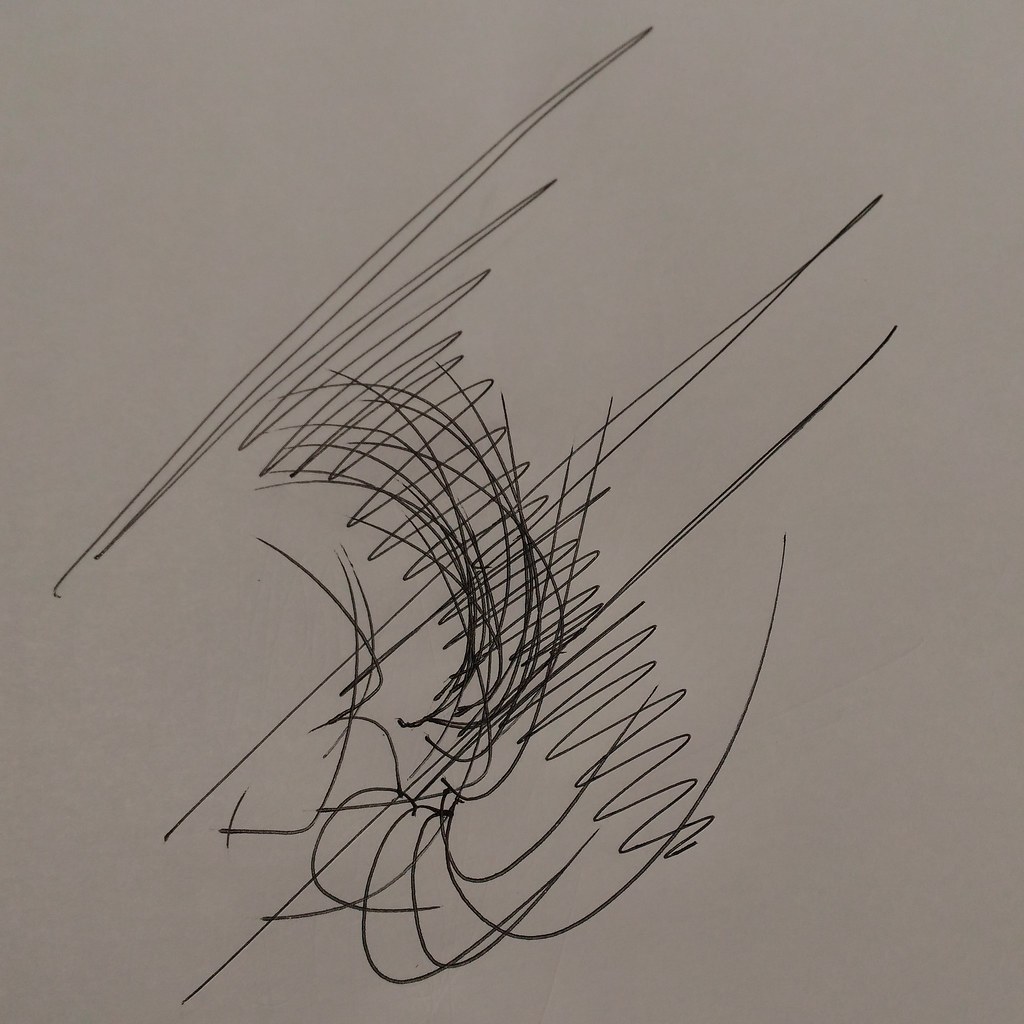The image is a detailed sketch made with a fine point black marker on a light lilac background, drawn within a square frame. The artist began near the upper left corner, leaving a small triangular area of empty space, before sketching a series of vertical, closely-spaced zigzag lines. These lines start from the left, extending diagonally up to the right, then back down, each time decreasing slightly in height and widening at various points. This repeated up-and-down pattern continues until it reaches approximately three-quarters of the way down the square.

Subsequently, the artist added about six swooping lines that form partial circles, overlaying the zigzag pattern. These swoops cascade in a rhythmic sequence, adding a dynamic contrast to the original zigzag lines. Lastly, several backward L-shaped scribbles are placed in the lower left section of the square. These L-shapes curve gently as they ascend towards the right, adding a subtle organic element to the overall composition.